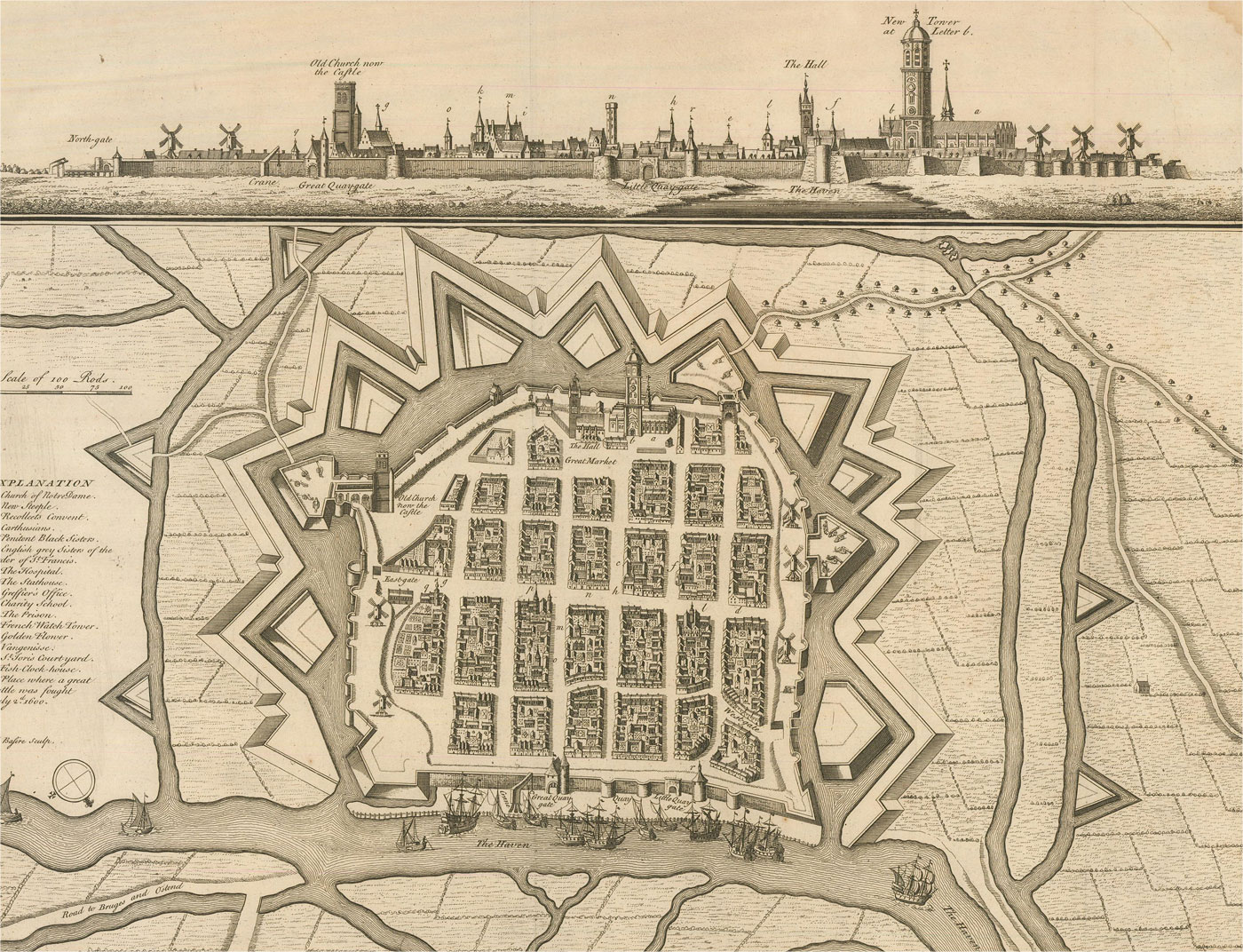This is a very old hand-drawn sketch on a yellowed piece of paper, depicting a medieval-style city enclosed by a prominent rock wall. The upper section of the image illustrates a landscape view from ground level, showcasing several churches and windmills, as well as a large building resembling a castle with tall spires and security towers spaced along the wall. One particularly high tower stands out among the structures. The foreground features water with boats, leading to a detailed overhead map of the area. This map outlines square plots of ground arranged in a geometric diamond pattern, resembling a grid formation which becomes irregular towards the edges. The sketch is predominantly black and white with some brown shading. Additionally, there is text on the left side and atop some of the towers, though it is not legible. The entire piece suggests a historical or cartographic representation combining both landscape and architectural elements.